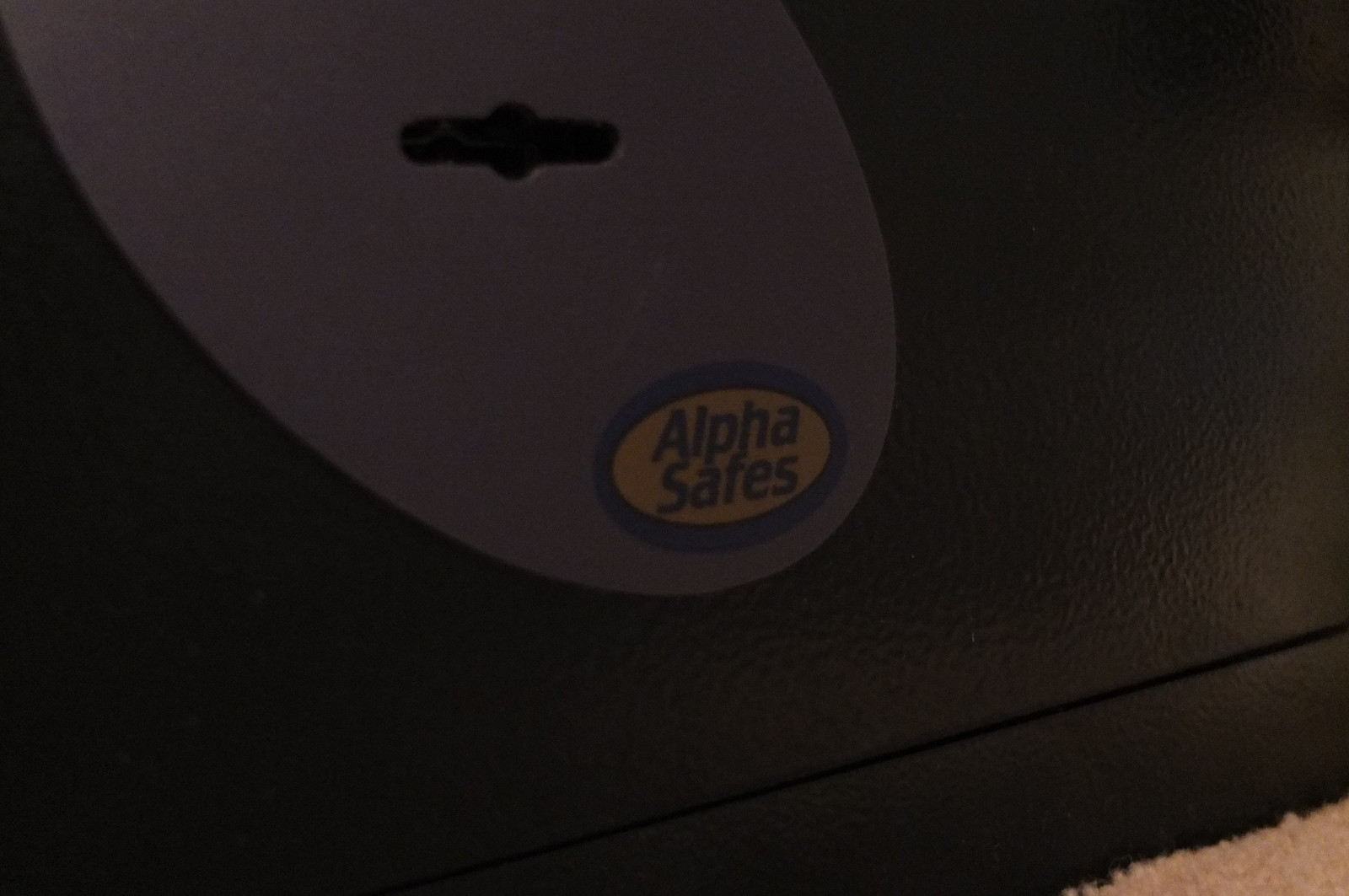This horizontal, rectangular image is largely enveloped in darkness, with a focus on the black, metallic side of a hotel-style safe. In the very bottom right corner, a small portion of light-colored carpeting is visible. Dominating the center of the image is an oval sticker with a yellow background and blue text, clearly bearing the words "Alpha Safes." This oval also contains a keyhole. The safe's surface and the sticker's details are the primary features, with the rest of the image remaining indistinct in the darkness.